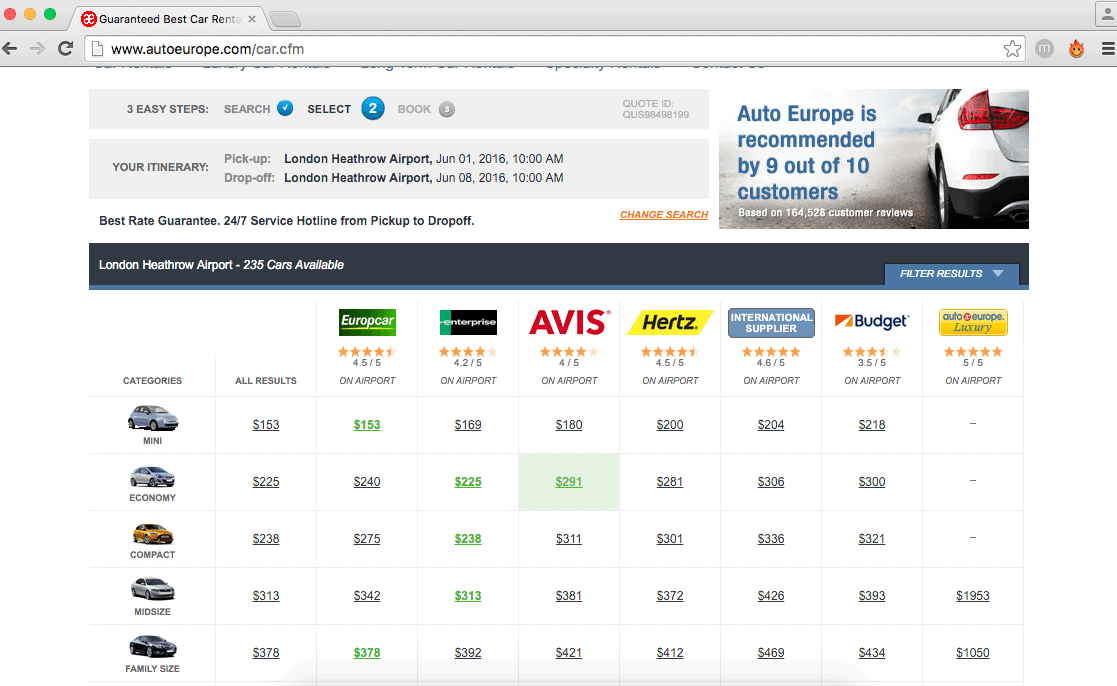This is a detailed screenshot of a browser window open to the website AutoEurope.com. The browser's top header is grey, featuring three small circular buttons in the top left corner colored red, yellow, and green. To the right of these buttons is the active tab, which displays an 'X' for closing the tab, "Guaranteed Best Car Rental," and the Auto Europe icon.

Directly below the tab area is the search bar, which includes a left-pointing arrow, a right-pointing arrow, and a refresh icon. The main content of the webpage has a white background and has been scrolled down slightly, cutting off the top portion of the page.

Within the visible section of the webpage, there are two primary boxes. On the left, a box outlines "Three Easy Steps: Search, Select, and Book." The "Search" and "Select" steps are already highlighted, while the "Book" step remains greyed out. To the far right of this, there is a quote ID displayed.

Below this, another grey box is labeled "Your Itinerary," detailing the pickup and drop-off locations, along with the corresponding dates set for the rental. Further down, there is a list of rental cars on the left, with corresponding prices to the right. This section includes seven columns, each representing different car rental companies along with their respective prices for each listed vehicle.